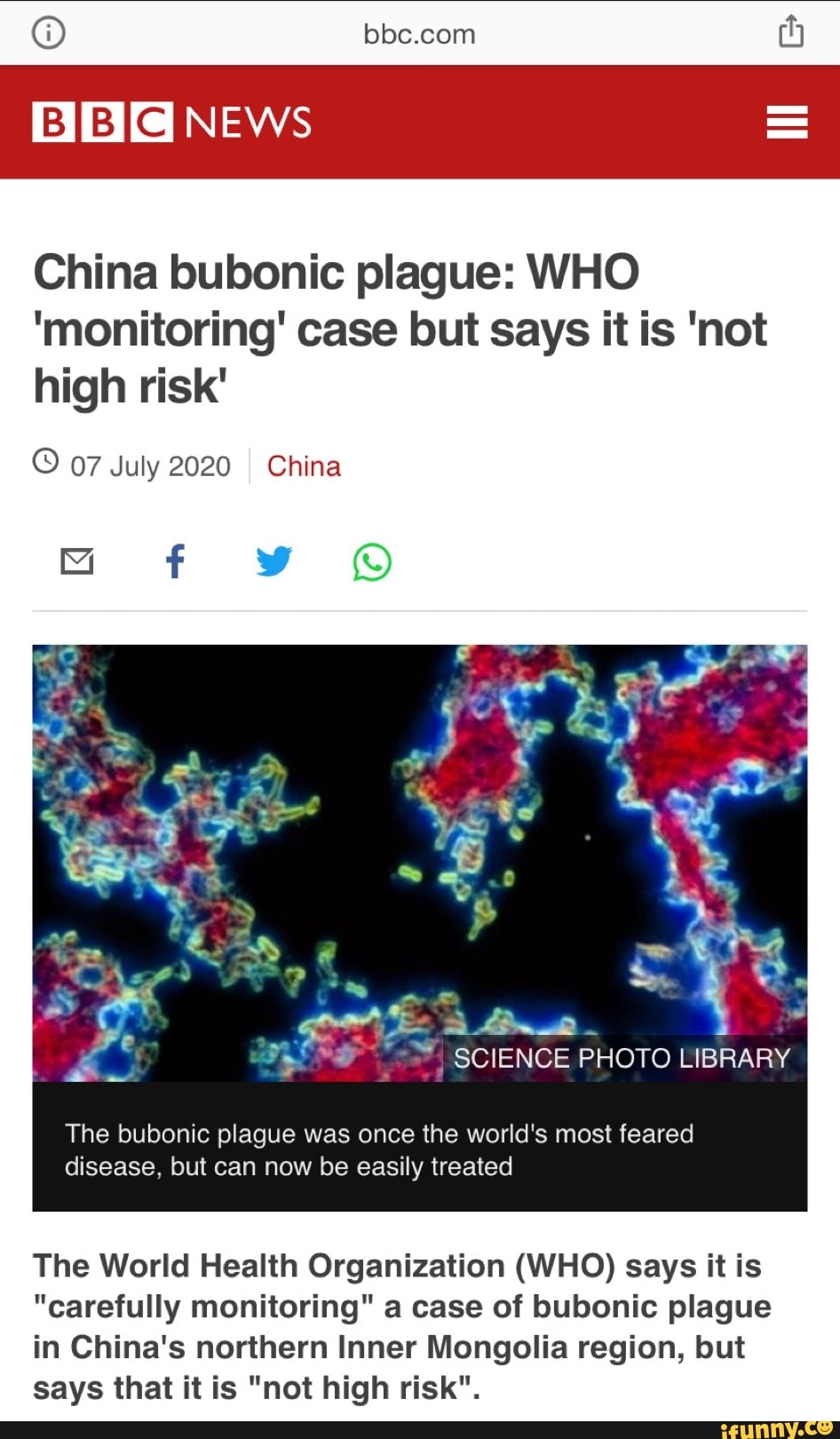The image depicts a webpage with the URL "bbc.com" prominently displayed in the header against a grey background with black text. Directly below the URL is a red banner with the text "BBC News" in white, positioned to the left, while an icon is situated on the right side of the banner.

Beneath the red segment, the main body of the page begins with a white background. The headline, written in black, reads: "China: Bubonic Plague case being monitored; WHO says it is not high risk." Adjacent to this headline, the details indicate the date "7 July 2020" and the location "China," where "China" is highlighted in red.

Further down, there are social media sharing icons: a grey mail icon, a blue Facebook icon, a light blue Twitter icon, and a green WhatsApp icon.

Below the social media icons, an image featuring black, green, and red hues is displayed. In the bottom right corner of the image, the credit "Science Photo Library" is noted. Accompanying the image is a caption that reads: "The Bubonic Plague was once the world's most feared disease but can now be easily treated."

At the very bottom of the page, additional text from the article reads: "The World Health Organization (WHO) says it is carefully monitoring a case of Bubonic Plague in China's northern Inner Mongolia region, but asserts that it is not high risk."

The footer of the webpage includes further text, and in the bottom right corner, the text "ifan.co.nl" is visible.